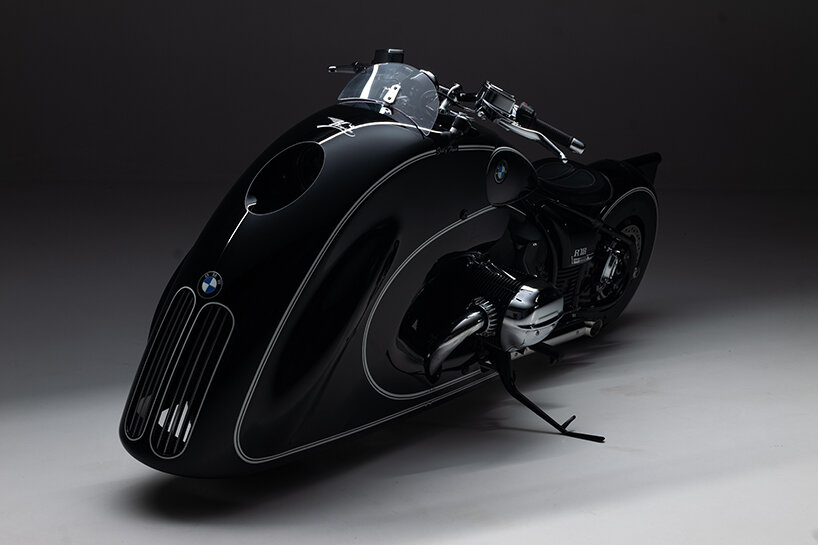This image features a sleek, futuristic motorcycle with a distinctive design reminiscent of a Batmobile. Unlike regular motorcycles, its front wheel is fully covered by an imposing black bumper, concealing the wheel entirely. Prominently displayed on the bumper is the iconic BMW logo, which is also visible on the side of the motorcycle. The logo features a circular design with blue and white quadrants, encased in a silver outline. 

The motorcycle itself is predominantly black, including its kickstand and handles, though it also boasts silver highlights on various components such as the pipes and the edges of a see-through windshield. The front portion of the bike has a prominent circular element at the top, flanked by cylindrical vents at the bottom, adding to its futuristic aesthetic.

The bike is in a parked state, supported by its black side stand, and is oriented facing towards the left. The back tire is visible, but the seat is not, suggesting a streamlined design. The engine, partially visible, features black and silver elements. The motorcycle design includes silver bars forming a grill at the front, contributing to its sophisticated look.

The background of the image consists of a gradient of grey, darker at the top and lighter at the bottom. The top wall is dark grey, blending into a lighter grey floor that starts from the bottom left corner and transitions towards the right side of the image. This nuanced background enhances the striking appearance of the motorcycle, making it stand out prominently.